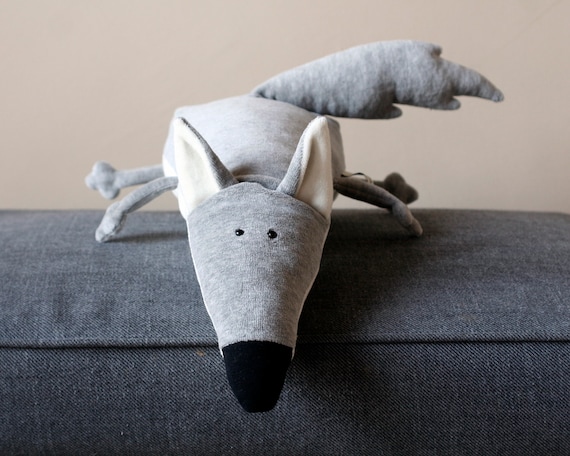This photograph captures a plush stuffed toy that resembles a playful, cartoonish dog, prominently centered on a dark green cushion. Its triangular, conical head is light gray, with two small, black beady eyes, and a pointed, black nose at the tip. Perched atop its head are two perked-up ears, gray on the outside and white on the inside, adding to its animated character. The stuffed dog has a fully gray exterior, including its four outstretched legs and thick, slightly wavy tail. The toy's bushy tail extends to the right, and it appears to be gazing straight at the camera. The background features a muted, beige or grayish wall that complements the overall subdued yet charming aesthetic of the image.